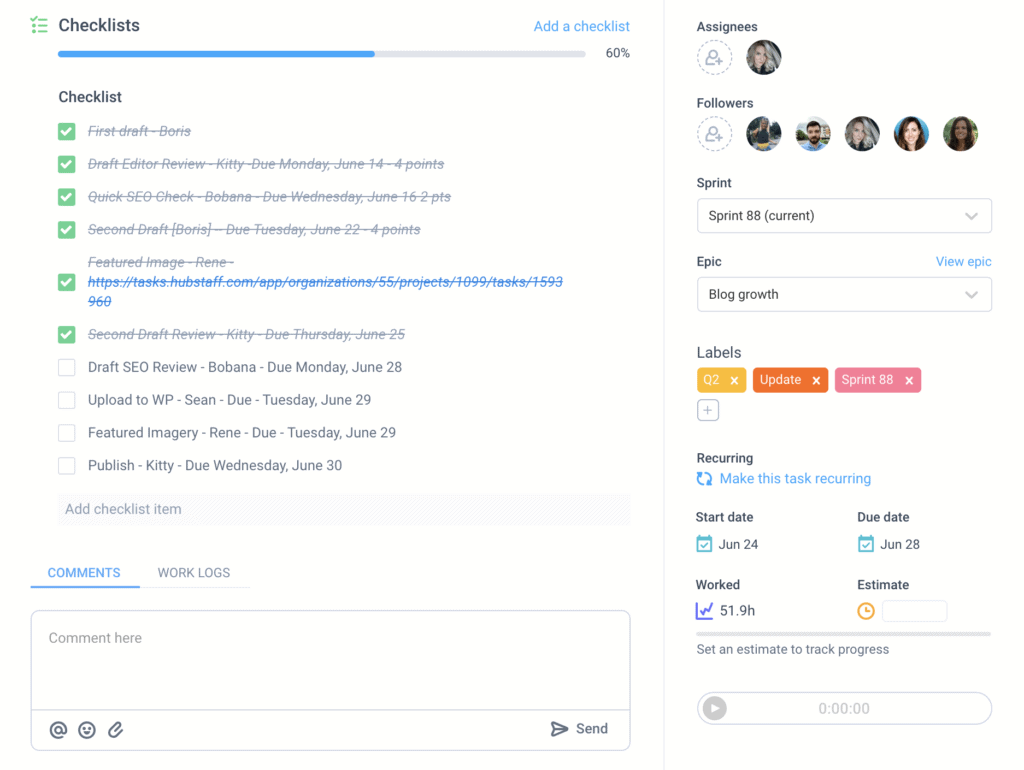The image depicts a detailed project management interface centered around a checklist that tracks the progress of various tasks. The checklist box indicates that the current completion level is at 60%, visualized with a progress bar halfway filled. To the left of the progress bar, a green emoji adds a touch of positive reinforcement. To the right, there is an option to "Add a checklist," allowing for the inclusion of additional checklists if needed.

Directly beneath the progress bar is a bolded checklist with several tasks, each checkmarked in green and struck through to signify their completion. The first task reads "First draft, Boris," marked as done with a green checkmark and a strikethrough. The next task is "Draft editor review, KD due Monday, June 14th," which earns 4 points. This is followed by "Quick SEO check, due Wednesday," worth 2 points, and is similarly checkmarked and crossed out. The "Second draft" task also appears twice, both times checkmarked and crossed out. Additional tasks that have yet to be completed include "Draft SEO review," "Upload to WP," "Featured imagery," and "Publish." Below this checklist, there is another option to "Add checklist."

Additionally, the interface features a comment section where users can leave comments, log their work, and attach files. To the right of these sections, there is an "Assignments" column displaying the current person assigned, illustrated with a profile picture of a girl. Five followers are also listed, indicating team members who are tracking the task.

The interface includes a "Sprint" dropdown box, currently set to "Sprint 88," that can be adjusted. An "Epic" dropdown appears next, labeled "Blog Growth," which is also adjustable. Three different labels are shown: a yellow label for "Q2 updates," an orange-pink label for Sprint 88, and a pink label.

Users can set tasks as recurring, establish a start and due date (June 24th to June 28th), log hours worked, estimate the time for task completion, and use the "Set an estimate to track progress" button to manage the progress effectively.